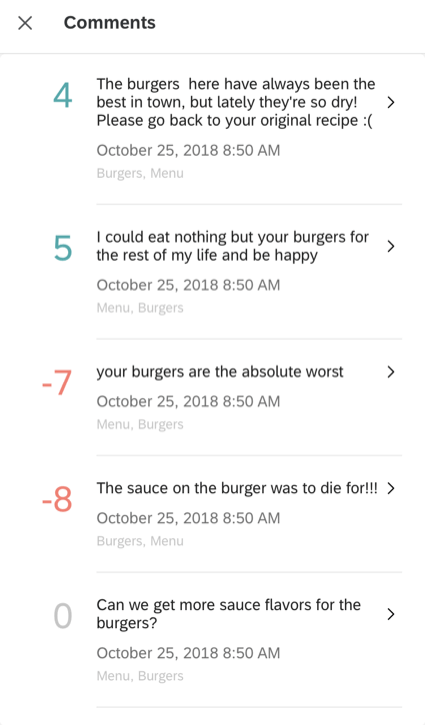This image is a screenshot displaying user comments on a webpage, with a sorting or voting feature indicated by numeric values in varying colors. 

In the top left corner, there's an "X" icon for closing the comment section. To its right, the label "Comments" is displayed. Below it, a teal number "4" signifies a vote count or ranking, followed by a comment in black text: 

"The burgers here have always been the best in town, but lately, they're so dry. Please go back to your original recipe from October 25th, 2018, at 8:50 a.m. - [burgers, menu]"

The next tier features a teal number "5" paired with the text:

"I could eat nothing but your burgers for the rest of my life and be happy - [October 25th 2018, 8:50 a.m., menu, burgers]"

Following this, an orange number "-7" precedes the comment:

"Your burgers are the absolute worst - [October 25th 2018, 8:50 a.m., menu, burgers]"

Below, an orange "-8" is shown next to:

"The sauce on the burger was to die for - [October 25th 2018, 8:50 a.m., burgers, menu]"

At the bottom, a gray "0" marks the final comment:

"Can we get more sauce flavors for the burgers? - [October 25th 2018, 8:50 a.m., menu, burgers]"